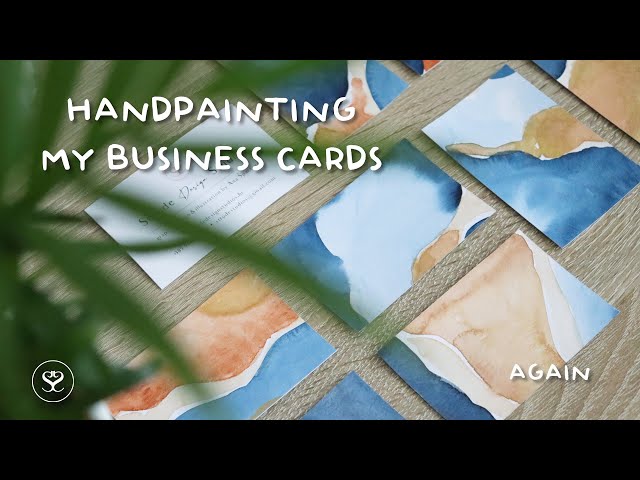This is a screen capture of a video titled "Hand Painting My Business Cards" with black borders on the top and bottom. The video still shows watercolor business cards laid out on a light wooden table, painted in shades of blue and orangey-brown. The camera artistically peers through a green plant, focusing on the cards' backsides. Partially visible is some blurred text. In the upper left corner, "Hand Painting My Business Cards" is written in a handwriting font, in capital letters. In the bottom left corner, there's a circular logo depicting two mirrored S-shaped symbols, resembling two snakes and forming a heart shape. The word "AGAIN" is prominently displayed in capital letters in the bottom left corner.